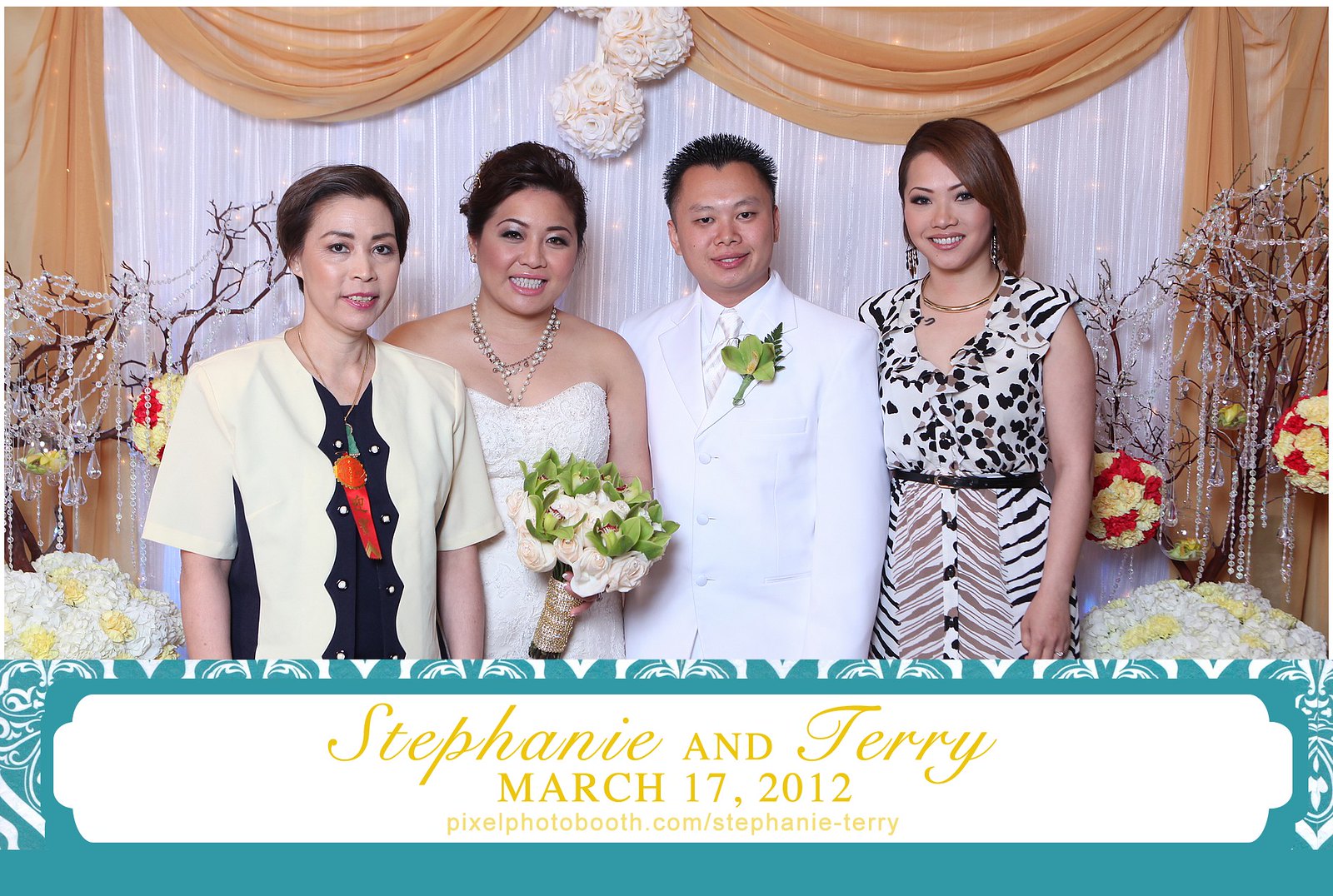This photograph, taken in a photo booth at a wedding, features a rectangular frame where the bottom 25% forms a teal-colored banner with a white rectangle in the center. Inside this white section, in gold cursive letters, it reads "Stephanie and Terry," with "AND" in all capitals. Below this, it states "March 17th, 2012" in sans-serif capital letters, followed by a URL: "pixelphotobooth.com/Stephanie-Terry."

The upper 75% of the image shows four people against a backdrop of white drapery with gold panels. The bride, positioned centrally, is wearing a white dress and is holding a bouquet of white and green flowers, with her hair pinned up and adorned with pearl necklaces. Beside her is the groom, also central, dressed in a white suit, shirt, and tie, accented by a green boutonniere on his left lapel. To the left stands an older woman in a black and white patterned dress with short brown hair. To the right, another woman has shoulder-length reddish-brown hair and is wearing a white, black, and brown patterned dress with a red accent in the center.